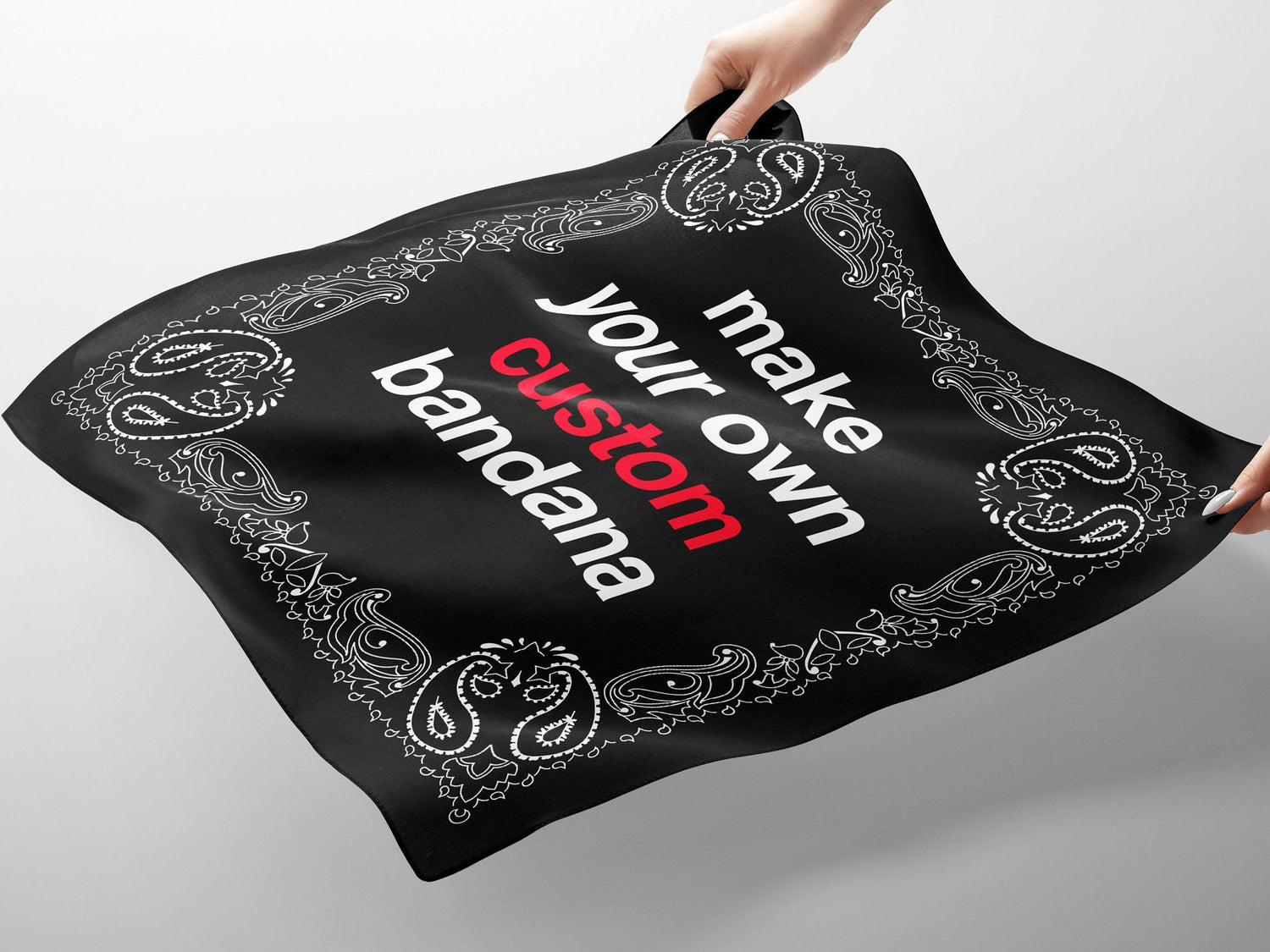In this advertisement, a black bandana with a white paisley pattern around its borders is prominently displayed against a grayish off-white background. A woman's hand with painted fingernails is holding the bandana in the upper part towards the right, stretching it flat and slightly angled. The design on the bandana is symmetrical, featuring a border with teardrop elements meeting in the corners and a floral-like motif. In the center of the bandana, bold white lettering reads "Make Your Own Custom Bandana," with "custom" standing out in red font. The background shows a darker gradient towards the bottom edges, likely due to the shadow cast by the bandana held above it.